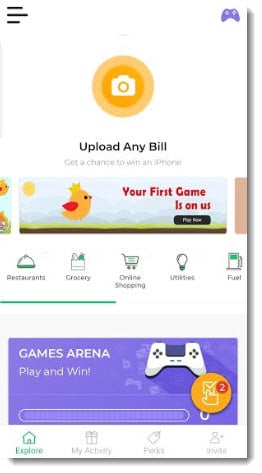Screenshot of a mobile application interface displaying a prominent yellow circle in the center with a camera icon inside. Below the circle, there's a text prompt that reads, "Upload any bill." Underneath, a small box contains the message, "Your first game is on us." Further down, there are various small categories listed, though the text appears somewhat tiny and less legible.